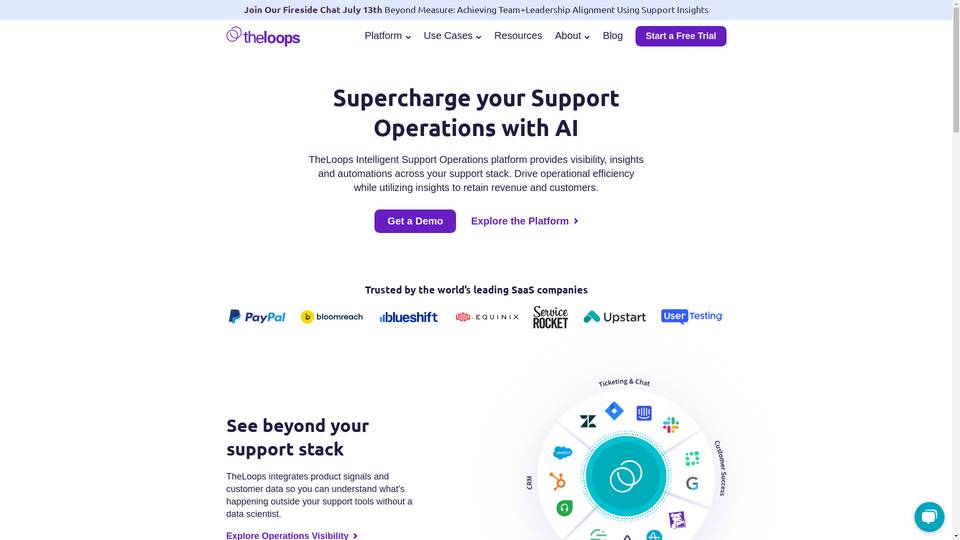Screen capture of a website showcasing various elements and features. On the left side of the image, a gray scroll bar is visible. The main content area features a thin blue strip at the top with a purple announcement reading, "Join Our Fireside Chat - July 13th: Beyond Measures - Achieving Team Leadership Alignment Using Support Insights." Below this header, the website displays a logo of two interconnected rings labeled "The Loops."

Further down, there are clickable navigation links in black with arrows: "Platform," "Use Cases," "Resources," "About," and "Blog." A prominent purple and white box invites visitors to "Start a Free Trial." In black text, the site promotes, "Supercharge your support operations with AI. The Loops' intelligent support operations platform provides visibility, insights, and automations across your support stack, driving operational efficiency while utilizing insights to retain revenue and customers."

Another purple and white box offers a "Get a Demo" option, while a purple button encourages visitors to "Explore the Platform." Trust seals from various companies are displayed, including "PayPal" (blue logo), "Blooming Tech" (yellow logo), "Blueshift" (blue logo), "Equinox" (red logo), "ServiceRocket" (black logo), "Upstart" (teal arrow logo), and "UserTesting" (blue logo). 

At the bottom of the page, black text reads, "See Beyond Your Support Stack. The Loops integrates product signals and customer data so you can understand what's happening outside your support tools without a data scientist." A purple button invites users to "Explore Operations Visibility." Additionally, there is a chart featuring various company icons in black, blue, green, pink, yellow, and orange. Nearby, a teal and white circular icon resembling a text message bubble is visible.